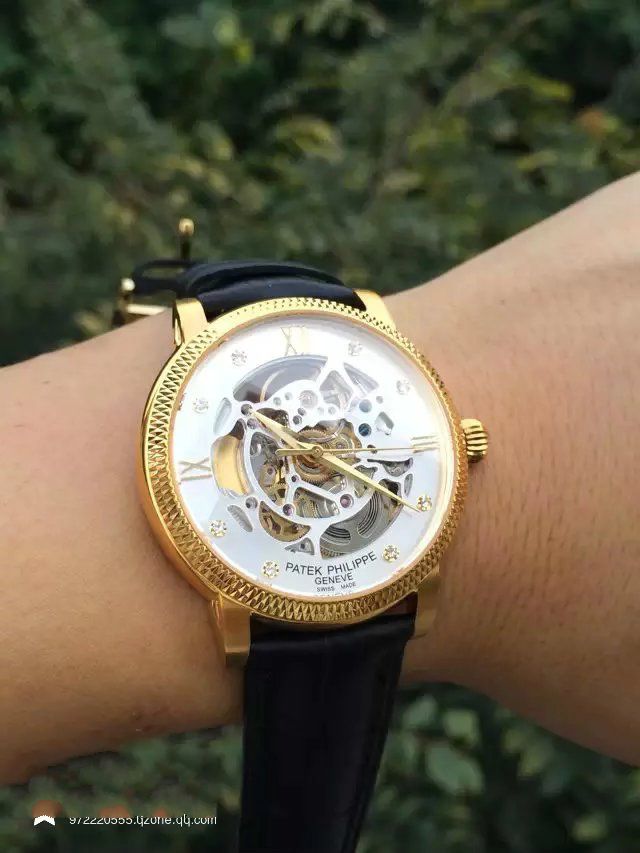This photograph features a wristwatch with a black leather strap draped over a Caucasian wrist, likely female. The wristwatch boasts an elegant golden frame and housing, complete with a gold circular knob on the side. The watch face is predominantly white but features a transparent central area that reveals intricate exposed gears, accentuating the timepiece's mechanical allure. Roman numerals mark some of the hours, while glimmering diamonds indicate the remaining positions. All three hands—the hour, minute, and second—are gold, complementing the watch's opulent aesthetic. The background of the image is filled with lush green foliage, adding a natural contrast to the sophisticated watch. Additionally, a partially visible website is seen at the bottom of the image.